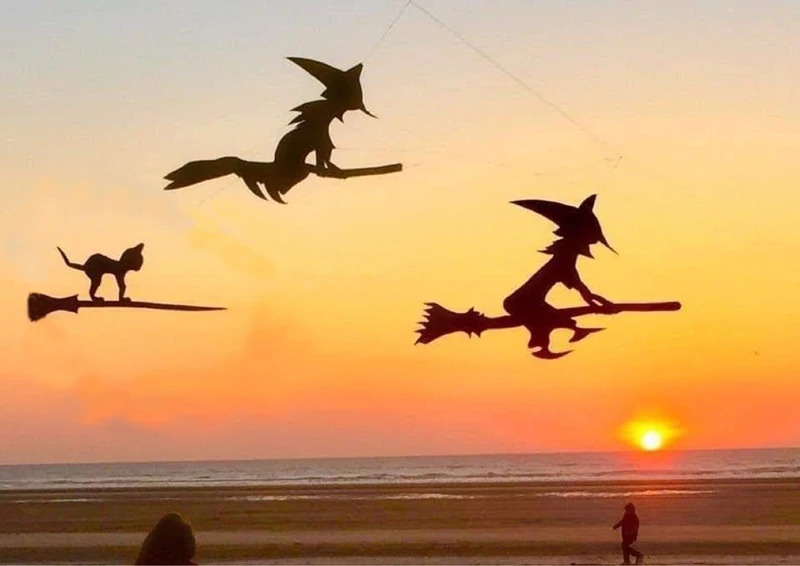The photograph captures a serene beach scene during a vibrant sunset or sunrise. The bottom fifth of the image reveals a stretch of sandy beach and gentle waves extending towards the horizon. The sky above transitions from rich orange and yellow hues to a light gray at the top, as the sun, a glowing sphere emitting yellow rays, hangs low in the right corner of the frame. On the left side, nearer to the horizon, we see the silhouette of a person walking on the beach, heading towards the left.

Dominating the sky in the top portion of the image are three whimsical kite silhouettes. These kites are creatively designed to resemble two witches and a cat riding on broomsticks, appearing as though they are flying. The witches, outlined in dark brown or black, face towards the right, while the cat, standing on its broomstick, follows behind. The silhouettes of these characters add a playful, magical touch to the tranquil seascape, their presence beautifully juxtaposed against the colorful, setting sun.